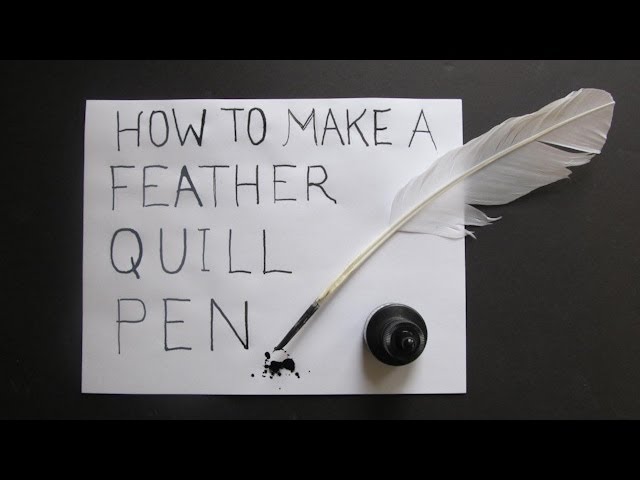A detailed photograph features a white sheet of paper placed against a gray backdrop. Prominently displayed on the paper are the words "How to Make a Feather Quill Pen." In the lower corner of the sheet rests a small bottle of black ink. Subtly placed above the ink bottle on the same paper lies a delicate white feather quill. The feather extends gracefully across the upper portion of the quill pen, culminating in a tip that is stained black, indicating it has recently been dipped in the nearby ink. Surrounding the tip are several fine spatters of black ink, adding a touch of artistic chaos to the otherwise orderly scene. The image is bordered by sleek black bands at the top and bottom, framing the composition perfectly.